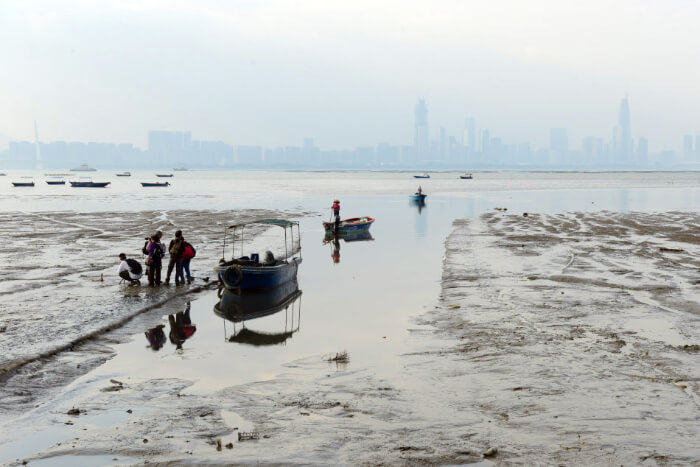This color photograph, taken in landscape orientation, captures a bustling bay scene set against a luminous city skyline. The horizon begins about halfway up the image, showcasing a silhouetted cityscape with tall skyscrapers bathed in shades of blue beneath a lighter blue and white sky. Below, the bay opens up with a mix of small fishing boats dotting the waterscape. Closest to the horizon, the boats appear as black silhouettes, while nearer to the viewer, a larger blue boat, covered with a tarp for shade, moves closer to shore. The shallow waters near the foreground feature a person dressed in red aboard another boat, adding splashes of color.

To the front left, a larger vessel is prominently beached in the muddy shoreline, angled towards the bottom left corner. This boat is in deep shadow, outlined in black, with a group of people disembarking onto the muddy terrain. These individuals, wearing red, yellow, and white, stand to the left of the boat, carrying bags on their backs. Their reflections, along with that of the blue boat, shimmer in a narrow channel that cuts into the sand and mud. Off to the right and further into the bay, additional boats float idly, hinting at a lightly anchored area. The beach and water merge into a muddy expanse with scattered puddles, capturing the scene's tranquil, albeit active, environment.